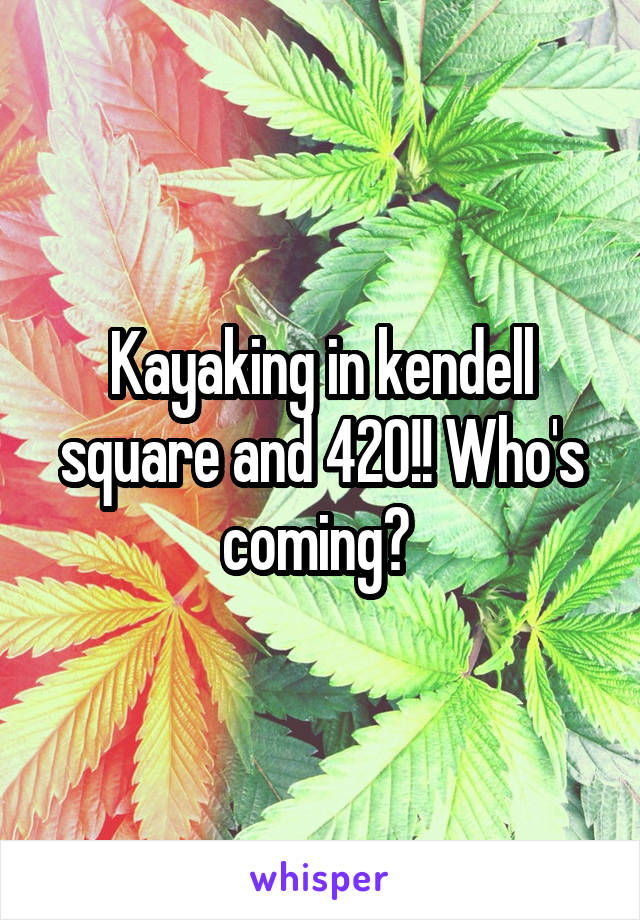This large vertical rectangular image is an advertisement styled like a meme, featuring vibrant marijuana leaves as the background. The background consists of variously colored marijuana leaves, including white, greenish leaves, green and white leaves on the right, and pink, white, orange, and white leaves on the left, which give a lively, multicolored impression. The leaves themselves vary in orientation, with some appearing flat and others standing up, adding depth and texture to the image.

In the middle of the poster, large white text outlined in black prominently reads: "Kayaking in Kendall Square and 420!! Who's coming?" This central text captures attention and makes the poster's invitation clear. Beneath this main text, the word "whisper" appears in lowercase blue or purple letters, suggesting a possibly discreet or intimate invitation, perhaps also indicating the name of the distributing entity.

The dark background behind the leaves enhances the contrast and depth of the image, making the vibrant leaves and bold text stand out vividly. Overall, this detailed description highlights the poster's announcement of a kayaking event in Kendall Square, infused with a playful reference to marijuana culture, and invites participants to join the fun.